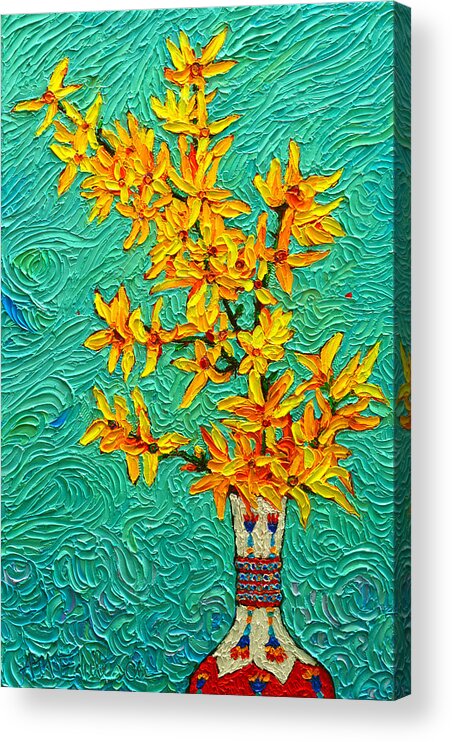The image is a vibrant and vividly colorful abstract painting, primarily dominated by bright yellows, reds, blues, and turquoise greens. **At the center of the image, a tall and skinny-necked vase is depicted, characterized by a red base and white neck with intricate blue and light blue patterns.** The vase houses **several flowers on long green stems, featuring thin, four-petaled bright yellow blooms sprinkled with subtle orange and red highlights, each flower centered with a dark spot**. 

**The background of the painting is teeming with dynamic textures and intricate details** reminiscent of an impressionistic style, showcasing the extensive use of thick oil paint strokes. The swirling, flowy background is a blend of greenish-blue and turquoise hues, evoking the sense of water or gas, enhancing the overall vibrant aesthetics. The entire artwork is framed within a large rectangular picture frame that is hung on a white wall.